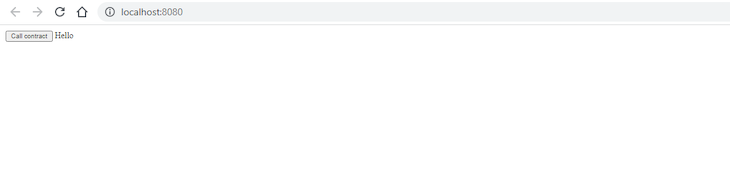The image depicts a mostly blank screen dominated by a vast expanse of white space. In the upper left corner, there is a browser toolbar featuring several light gray and black icons including a back button, a forward button, a reload button, and a home button. The URL bar, shaded in light gray, contains the address "localhost:8080" accompanied by an information icon represented by a lowercase "i" within a circle.

Beneath the URL bar, a faint horizontal light gray line spans the width of the screen. Positioned in the upper left section below this line, there is a button labeled "CALCONTRACT" (possibly representing "Cal Contract"). Next to the button, the text "hello" is typed out in lowercase letters. The remainder of the image is empty, highlighting the absence of any additional elements or content on the screen.